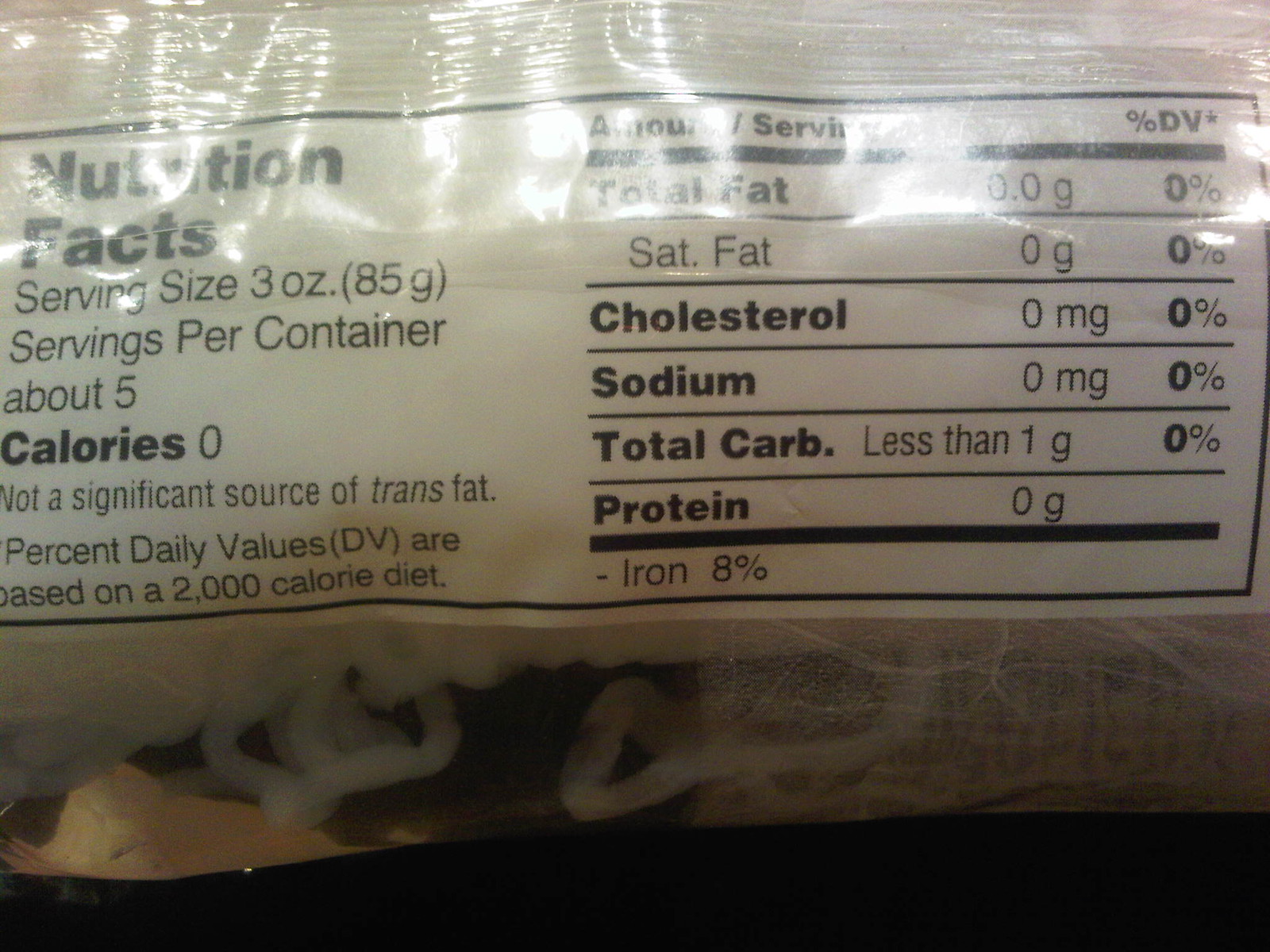A clear plastic package containing what appears to be fine, white noodles rests on a dark surface. The package's label is prominently displayed, featuring detailed nutrition facts. Each serving size is 3 ounces or 85 grams, with approximately 5 servings per container. The notably low-calorie content highlights 0 calories per serving. Additional nutritional details include 0 grams of total fat, cholesterol, and sodium; less than 1 gram of total carbohydrates; 0 grams of protein; and 8% of the daily recommended iron intake. The percent daily values are calculated based on a standard 2,000-calorie diet, emphasizing the product's health-conscious attributes.